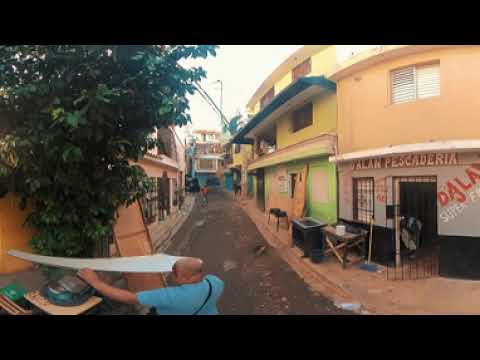This image captures a bustling downtown alley, likely in a Latin American country, characterized by colorful stucco buildings and a lively street scene. On the left side of the alley, a large, vibrant tree with lush green leaves stands in front of a row of attached orangish-red stucco buildings. A bald man with light brown skin is visible from the upper chest up, wearing a light blue short-sleeve t-shirt and a crossbody bag. He appears to be handling a piece of plywood or covering something on a white surface next to a table.

The narrow alley is lined with colorful, slightly run-down buildings. The structure closest to the viewer on the right features a gray and black ground floor and an eye-catching sugar-orange second floor. Above this, signage reads "Alan Pescaderia," suggesting a fish market or restaurant. The sidewalk in front of it is orangish-red, consistent with the predominant color palette of the alley. Towards the back, the upper levels of another building are painted yellow with lime green walls below, and a blue awning extends over a window. The scene is captured in daytime, with a clear sky overhead, adding natural light to the vibrant but somewhat downtrodden street. The presence of litter scattered across the road further adds to the sense of an area rich with everyday urban life.